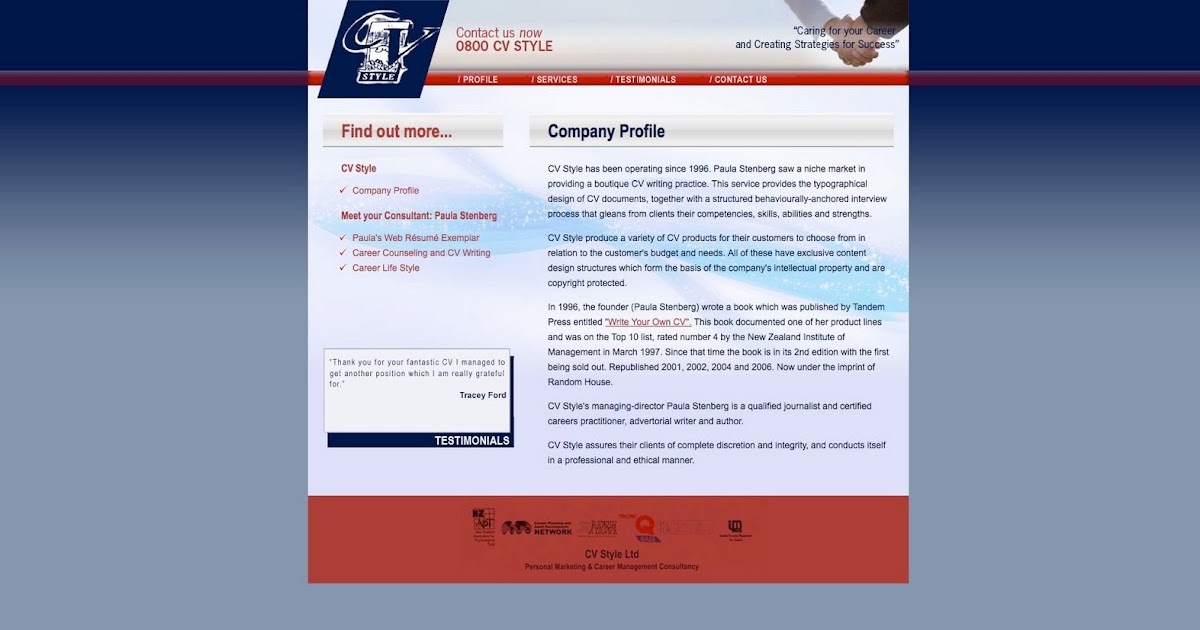A rectangular image primarily features a gradient background transitioning from blue at the top to light blue at the bottom. The layout is bordered at the top by a red banner containing white text. Within this central section, located on the far left, there is a blue rhombus-shaped box bearing the text "CV Style" accompanied by a relevant symbol. 

Moving rightward, bold red text commands attention with the message "Contact Us Now 0800 CV Style." On the extreme right side, an image of two hands shaking is partially obscured by illegible text due to its small size. 

The upper red banner hosts white text listing various sections: "Profile," "Services," "Testimonials," and "Contact Us." Below this, on the left side of the image, there is a prompt reading "Find Out More." Adjacent to this prompt is a column titled "CV Style Company Profile." Beneath this title, the text introduces "Meet Your Consultant Paula Stamberg." Additional points are listed below, but are too small to discern clearly.